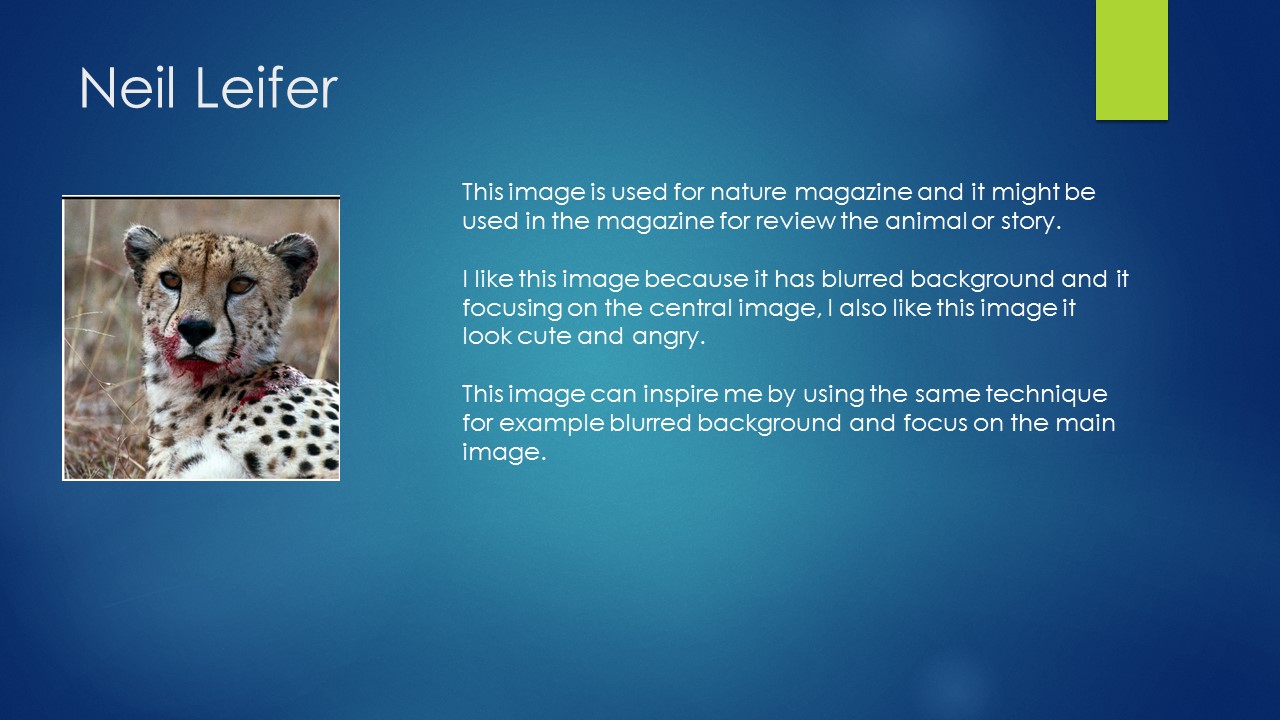The image presents a slideshow slide with a predominantly blue background that transitions from light blue in the center to darker blue at the edges. In the upper left corner, in white text, the name "Neil Leifer" is displayed. Below this text, there is a striking square photograph of a cheetah with blood on its mouth and fur, showcasing its distinctive spotted pattern and golden eyes. The photograph is set against a blurred grassland background, drawing sharp focus to the cheetah itself. To the right of the image, white text explains that the image is used for Nature Magazine and might be featured to review the animal or its story. The description highlights the photographic technique used, with a blurred background emphasizing the main subject. Additionally, a short lime green strip can be seen in the upper right corner of the slide, adding a subtle design element. Overall, the image draws attention for its vivid detail, emotive depiction of the cheetah, and the effective use of photographic techniques.